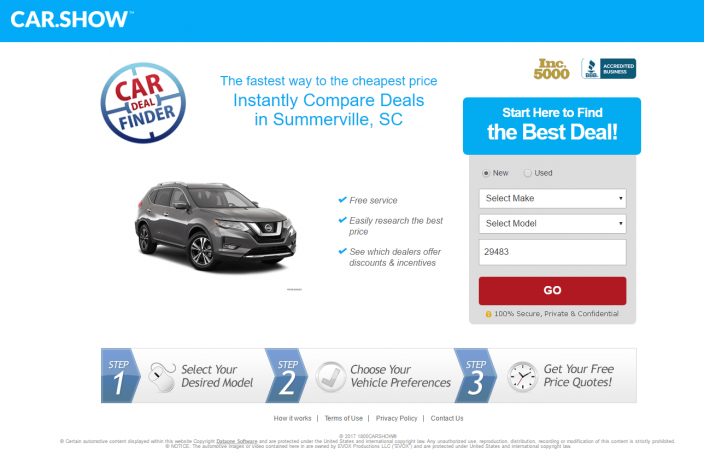A vibrant screenshot from the website Car.show features a sleek, professional layout with a light to baby blue banner across the top. In the top left corner, "CAR.SHOW" is prominently displayed in bold, white capital letters. Dominating the center of the page is a striking circular emblem labeled "Car Deal Finder," accompanied by the tagline, "The fastest way to the cheapest price. Instantly compare deals in Somerville, South Carolina."

To the right of this central feature, there is a proud display of the "Inc. 5000" designation next to the Better Business Bureau logo, signifying that the platform is an accredited business.

A dark gray, almost silver, SUV—likely a Nissan—captures attention beneath this main section. Beside the vehicle, a series of reassurances appears: a check mark next to "Free service," another next to "Easily research the best price," and a third indicating "See which dealers offer discounts and incentives." Below, a call to action encourages users with, "Start here to find the best deal," allowing selections for new or used vehicles, make, model, and a specific zip code for purchase location, culminating in a prominent "Go" button.

Further down, the site lays out a straightforward three-step process: 
1) Select your desired model
2) Choose your vehicle preferences
3) Get your free price quotes 
illustrated by a clock icon next to the final step, highlighting the efficiency and ease of obtaining the best vehicle deals.